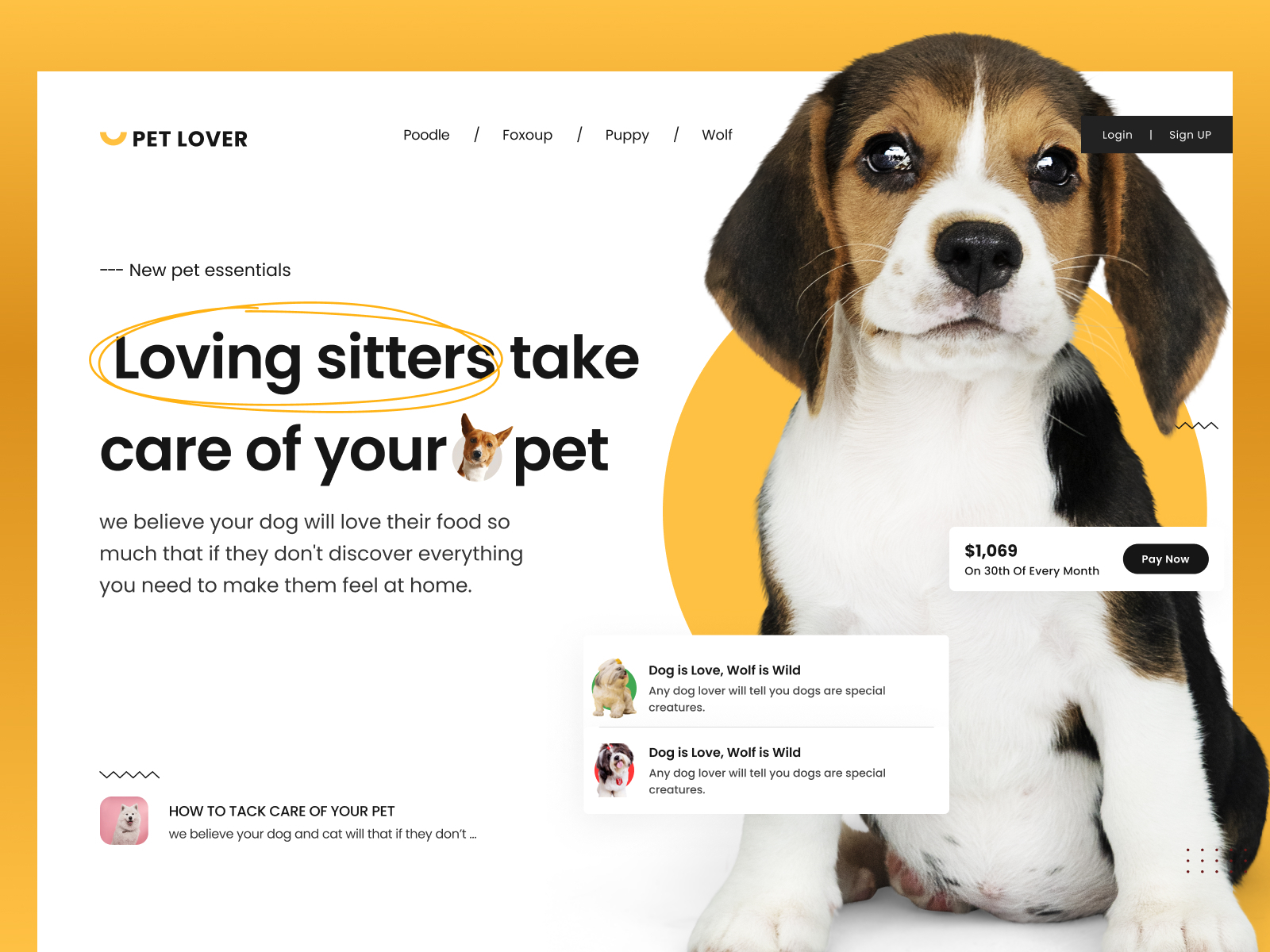In the image, there is a web page titled "Pet Lover" displayed prominently. The web page has a white background, and it is framed by a striking orange border along the top and sides.

On the left side of the web page, the heading "New Pet Essentials" is displayed. Just below this heading, key phrases such as "Loving Sitters" enclosed within an orange circle and "Take Care of Your Pet" are visible. Further down, there is a text block stating, "We believe your dog will love their food so much that if they don't, discover everything you need to make them feel at home." There is an additional instructional segment titled "How to Take Care of Your Pet," repeating the message about the assurances of pet satisfaction.

On the right side of the page, there is a top section featuring the navigation options "Login" and "Sign Up," both set against a black background. Immediately below is a vertical list of pet-themed content including "Poodle," "Foxoup (F-O-X-O-U-P)," "Puppy," and "Wolf."

Further down the right side, there is a bold statement, "Dog is Love, Wolf is Wild," emphasizing the unique qualities of dogs and their special place in the hearts of pet lovers. This message is duplicated just below. Additionally, a price tag displaying "$1,069" appears with a note indicating this amount is due on the 30th of every month, accompanied by a "Pay Now" button.

At the bottom right, there is an image of a beagle viewed from the front, adding a charming visual element to the page.